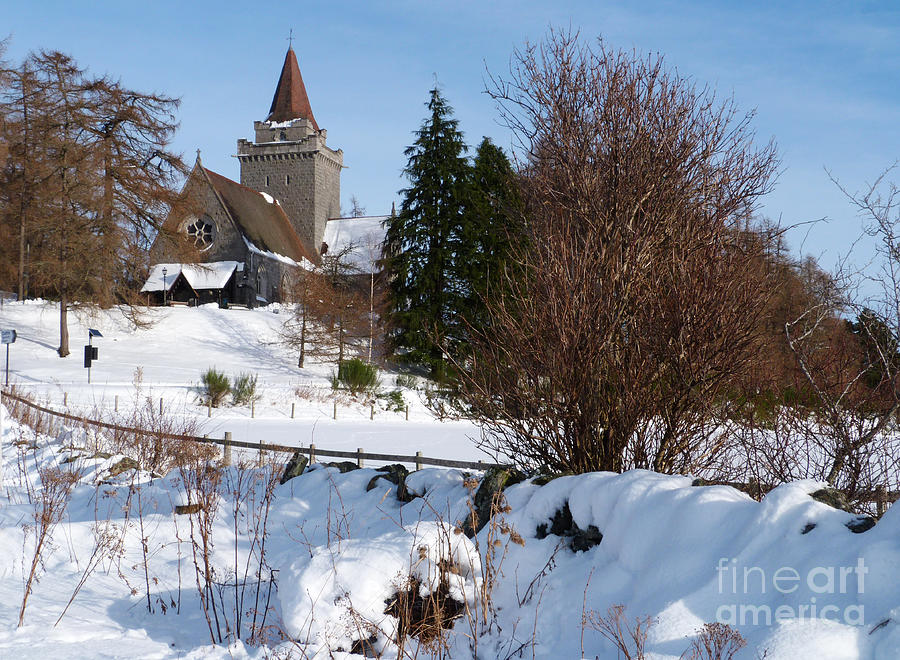In this wintertime outdoor scene, a photograph from "Fine Art America" showcases a serene, snow-covered landscape. Dominating the image is a brownish beige church, with its striking steeple topped by a metal cross. The building features a triangular front and a tower with a pointed roof, accentuated by a circular window. To the right of the church and partially obscured by its roof are two green pine trees, while additional pine trees with brown leaves are visible to the left. The church is framed by a wooden fence in the foreground, laden with snow, and surrounded by bare trees and twiggy plants indicative of the dormant season. The entire ground and rooftops are blanketed in pristine white snow, contrasting vividly with the clear blue sky above.